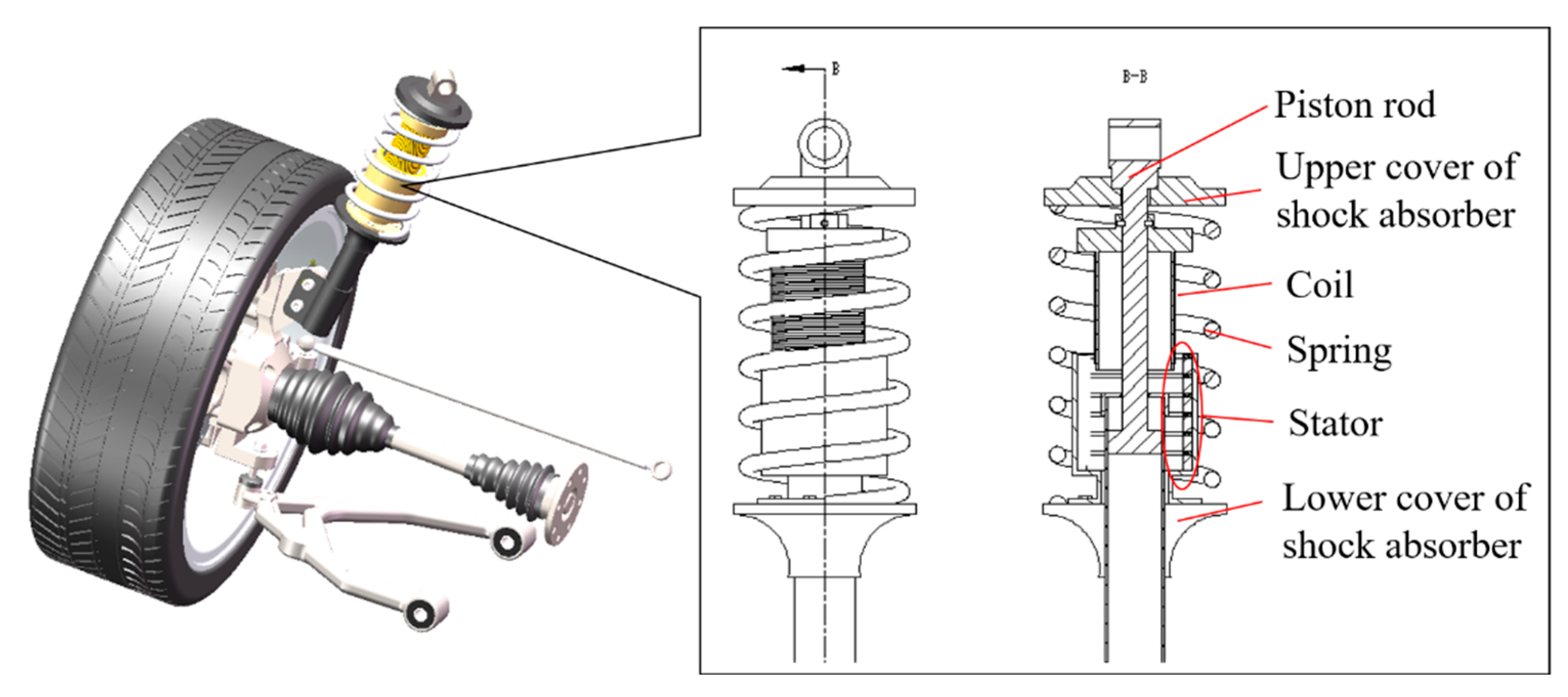The image is a detailed and instructional diagram of a car's wheel and its shock absorber assembly. On the left side, there is a photorealistic depiction of a black tire mounted on a wheel, with the axle extending from its center. Attached above the axle is a shock absorber which prominently features a yellow middle section. Several other machinery components are visible around the wheel, although they are not explicitly labeled.

The right side of the image presents a comprehensive breakdown of the shock absorber's internal structure through a black and white cross-sectional illustration. The diagram includes red annotations pointing to key parts of the shock absorber: the piston rod, the upper cover of the shock absorber, the coil, the spring, the stator, and the lower cover of the shock absorber. This annotated section aims to instruct viewers on the various components and their functions within the shock absorber system, ultimately guiding them on how it facilitates the tire's attachment and functioning.